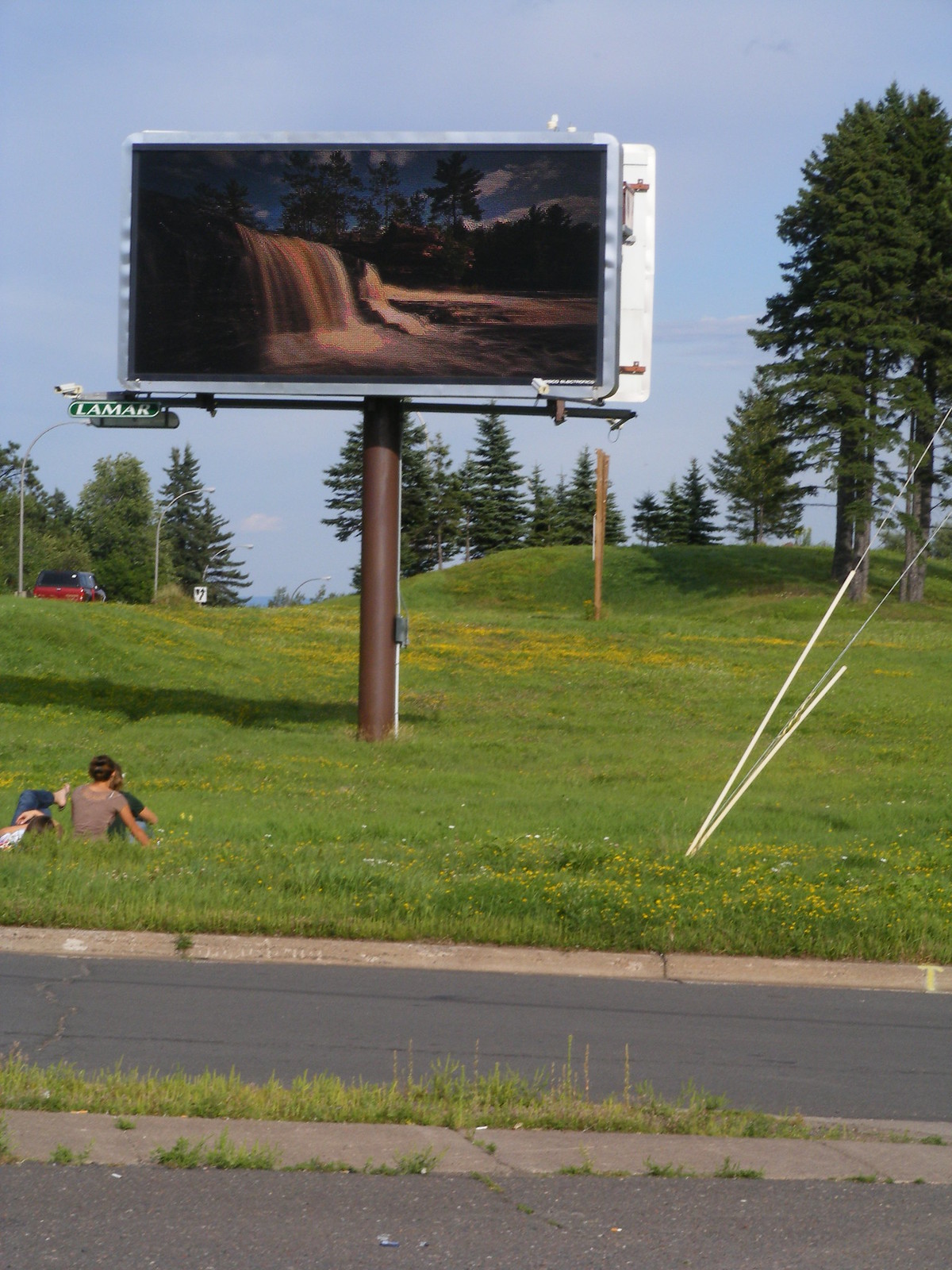This picturesque image captures a serene roadside verge adjacent to a narrow, single-track road. Stretching out from the road is a verdant expanse leading up to a gently sloping grassy knoll. In the foreground, several people are seen relaxing on the ground, either sitting or lying down, enjoying the tranquil setting. Dominating the center of the image is a large, live electronic notice board, vividly displaying an animated scene of cascading waterfalls with lush trees in the background. Behind this digital display, a dense cluster of towering pine trees adds to the natural beauty of the area. In the top left corner, a vehicle is visible, hinting at the presence of the road. Additionally, the scene is punctuated by safety measures; electrical wires, possibly for the notice board, are secured with visible white markers to prevent anyone from accidentally walking into them. The combination of natural elements and modern technology creates a unique and captivating landscape.